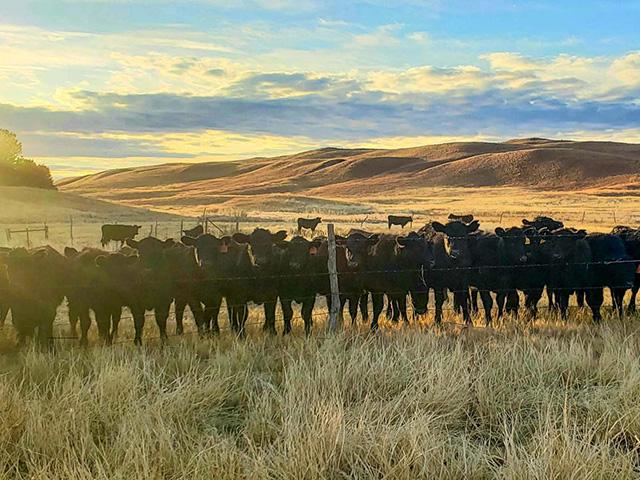In this striking image, a large group of dark brown cows line up along a weathered barbed wire fence, their gaze fixed intently on the photographer standing on the other side. The field in which they stand is covered in tall, dry grass with shades of yellow and green, stretching out under a vast, bright blue sky peppered with thick white and gray clouds. The sun, positioned just out of the frame, casts a radiant glow that slightly fades the left side of the photo, indicating late afternoon light. Behind the fence, more cows can be seen wandering in the background, dispersed across a broad, open expanse. The landscape is framed by gentle, rolling brown hills interspersed with sporadic trees, adding depth to the composition and enhancing the serene yet rugged rural scene.